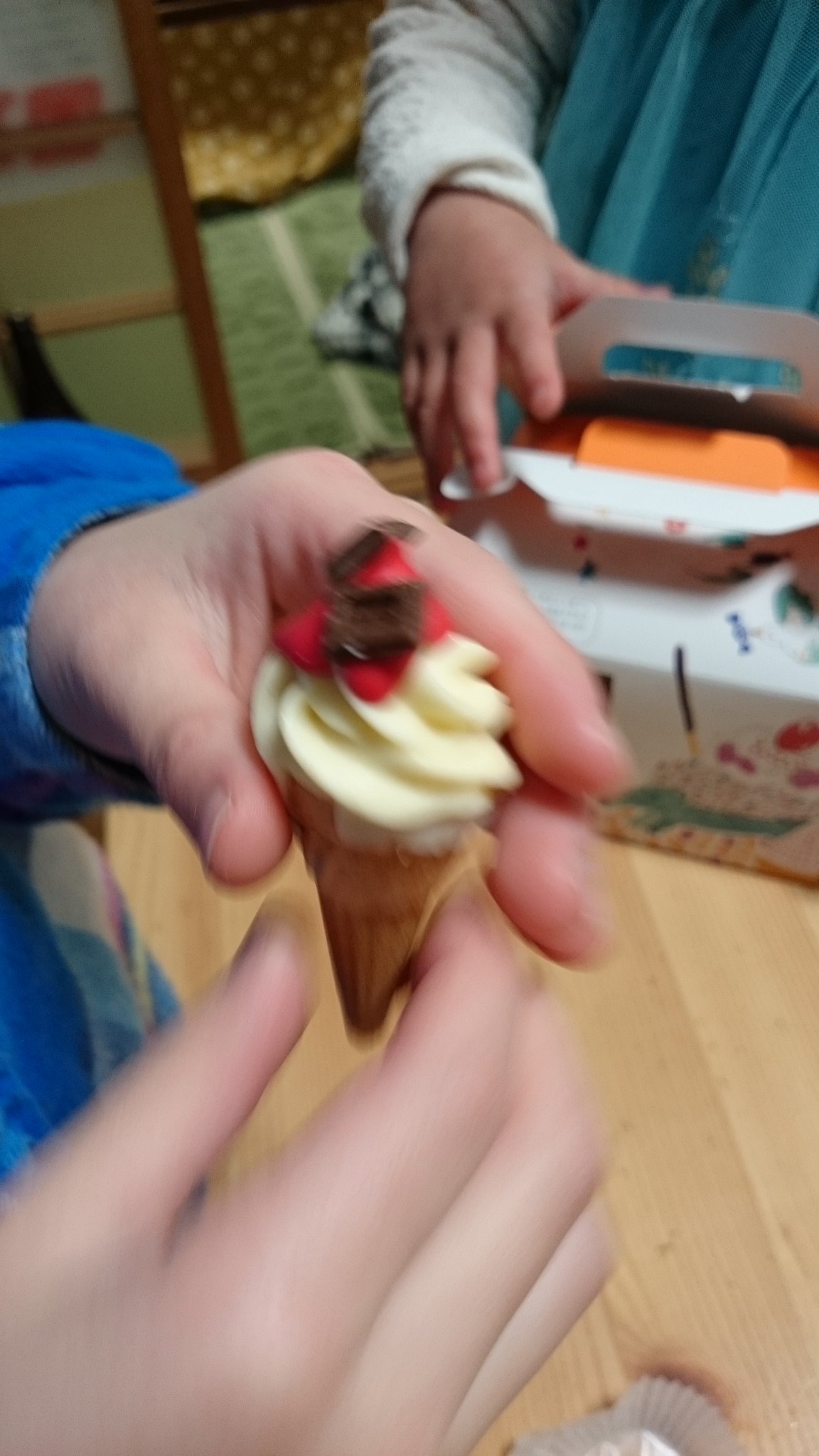This vertically cropped, slightly blurred color photograph captures a moment of casual interaction, likely taken during a birthday celebration or snack time at a kindergarten or preschool. The image showcases the torsos and hands of two individuals. On the left, prominently occupying the bottom two-thirds of the frame, a person in a blue shirt holds a small, white ice cream cone adorned with strawberry and chocolate toppings. This person is positioned above a round wooden table.

On the right-hand side of the table, a cupcake wrapper is visible, hinting at the presence of other sweet treats. Centrally, towards the left, a box of what appears to be donuts rests on the table. A young girl, identified only by her outstretched hand, reaches for the box, adding a dynamic sense of action to the image. The background subtly reveals a wooden floor and some other indistinct wooden object, contributing to the casual, informal atmosphere of the setting.